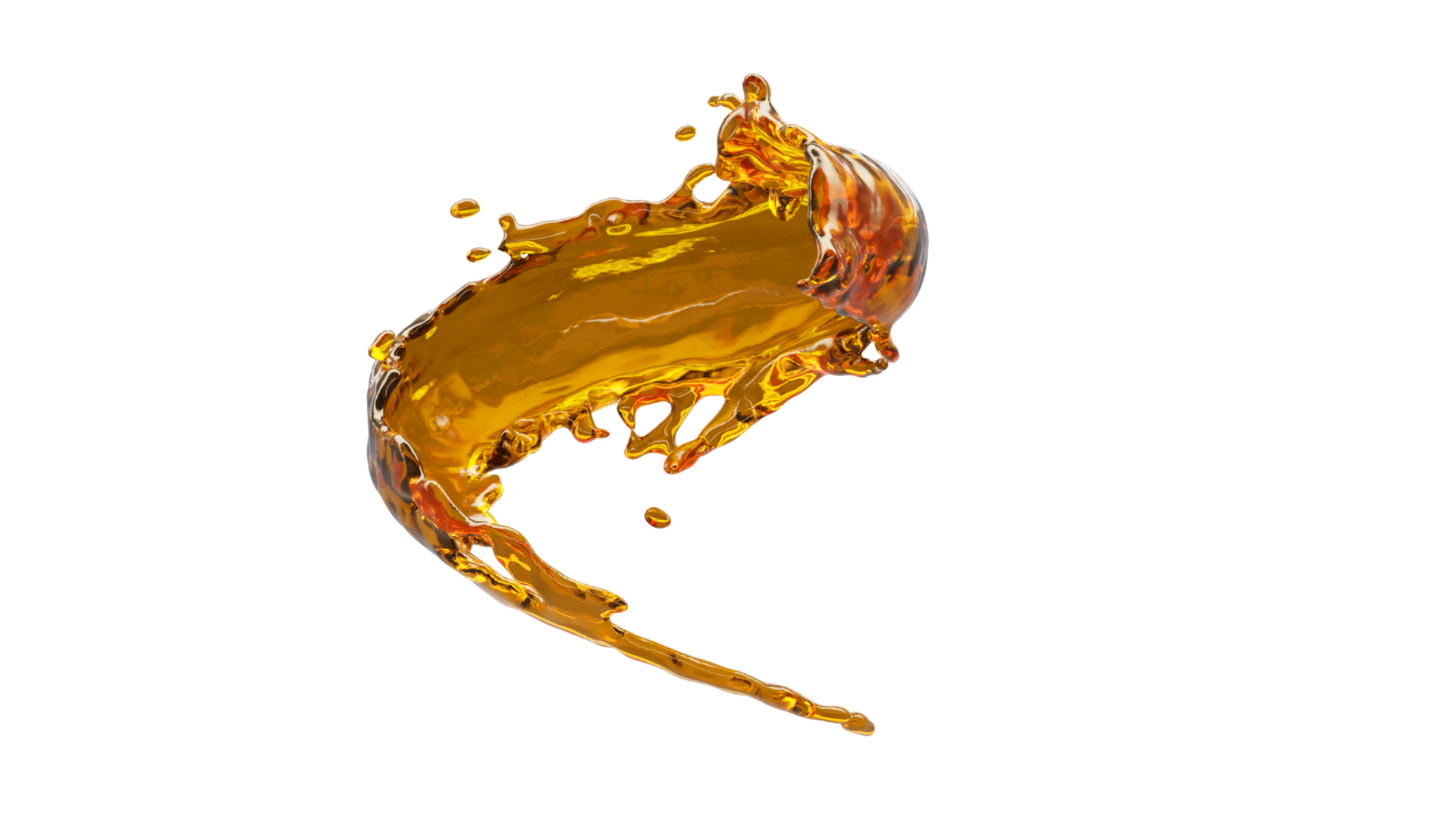The image depicts a striking, detailed portrayal of golden-yellow liquid captured in mid-motion against a completely white, featureless background. This swirling liquid, reminiscent of a boomerang or swoosh, has a dynamic curvature with a larger, concentrated mass at the top and tapering off towards the bottom, where smaller droplets begin to separate. The composition of the liquid reveals subtle tinges of orange and hints of brown, creating a captivating play of colors that enhance the visual impact. The liquid's swirling motion and intricate detail suggest it might be computer-generated or a meticulously captured photograph, frozen in time to highlight the fluid's graceful and kinetic form.